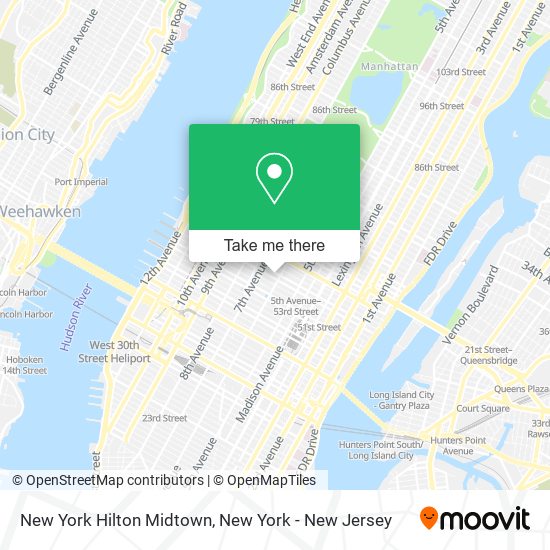This image features a detailed OpenStreetMap with multiple annotations and highlights. At the bottom, the credits read "OpenStreetMap contributors" and "OpenMapTiles." In the bottom left corner, in black text, it reads "New York, Hilton, Midtown New York, New Jersey." On the bottom right, the name "Moovit" is displayed in black text, with an orange location pin icon to the left of the letter "M."

The central focus of the map highlights a tall building with the text "Take me there" in blue positioned underneath it. The map itself shows prominent locations and streets such as Lexington Avenue and Madison Avenue. The Hudson River is identified on the left side of the map in blue, and FDR Drive is noted along with Beacon Line Avenue towards the top left. 

The map uses a distinct color scheme for various elements: blue for the river, yellow for main roads, white for the streets, gray for the buildings, and green for areas of vegetation.